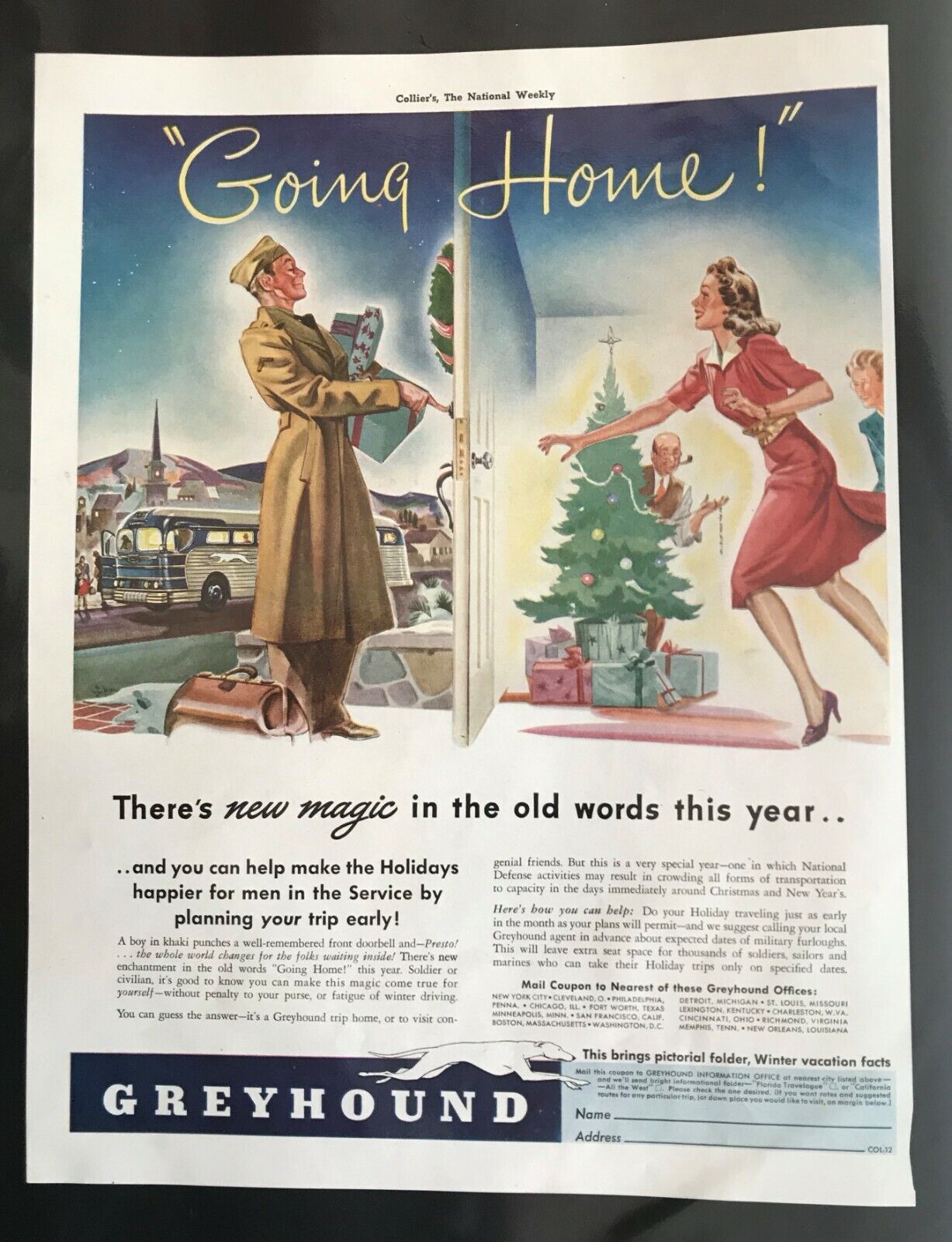The image presented is an old advertisement, likely from a 1950s issue of Collier's The National Weekly, for Greyhound bus services. The poster features a detailed illustration with a black border. The background of the poster is predominantly white, accentuated by vibrant colors in the illustration. The top of the poster displays the title "Going Home" in yellow letters.

On the left side of the illustration, a World War II-era soldier, identifiable by his cap and trench coat, stands at a house's front door, poised to press a doorbell. He carries presents in his left hand, and a leather bag rests at his feet. Behind him, a Greyhound bus and some buildings are visible under a blue sky, symbolizing his journey home.

On the right side, a festive scene unfolds inside the house, visible through a cross-section view. A woman in a red dress and high heels runs towards the door, her right hand extended to open it while her left hand is raised in excitement. Behind her, a decorated Christmas tree stands, and a man with a cigar or pipe peeks out from behind the tree. A child is also seen, seemingly curious about the visitor.

Below the illustration, the text reads, "There's new magic in old words this year," followed by a line encouraging viewers to help make the holidays happier for servicemen by planning their trips early. The Greyhound logo and a cut-out coupon offering a pictorial folder with winter vacation facts are featured at the bottom of the poster, reinforcing its purpose as an advertisement for Greyhound bus services.